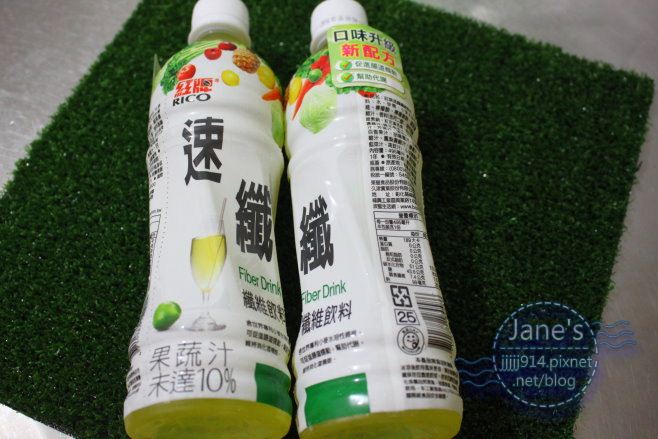This photograph features two identical 16-ounce plastic bottles of a fiber drink, each adorned with white caps and predominantly white labels. The labels showcase Japanese or Chinese characters, with "Fiber Drink" prominently displayed in green lettering. Through the partially transparent base of the bottles, a greenish, lemon-lime colored liquid is visible. The front of each label depicts a wine goblet filled with the green liquid, complete with a straw, and a lime positioned to the left of the goblet. Additionally, the label includes small images of various fruits such as peppers, pineapples, and lemons, suggesting potential ingredients. An inscription indicates "Rico" and there's a watermark mentioning "Jane's" along with a repeated URL www.jjjjj914.pixma.net. These bottles are pictured resting on a square of AstroTurf, which lies on a whitish linoleum floor, giving the entire scene an artificial yet colorful backdrop.